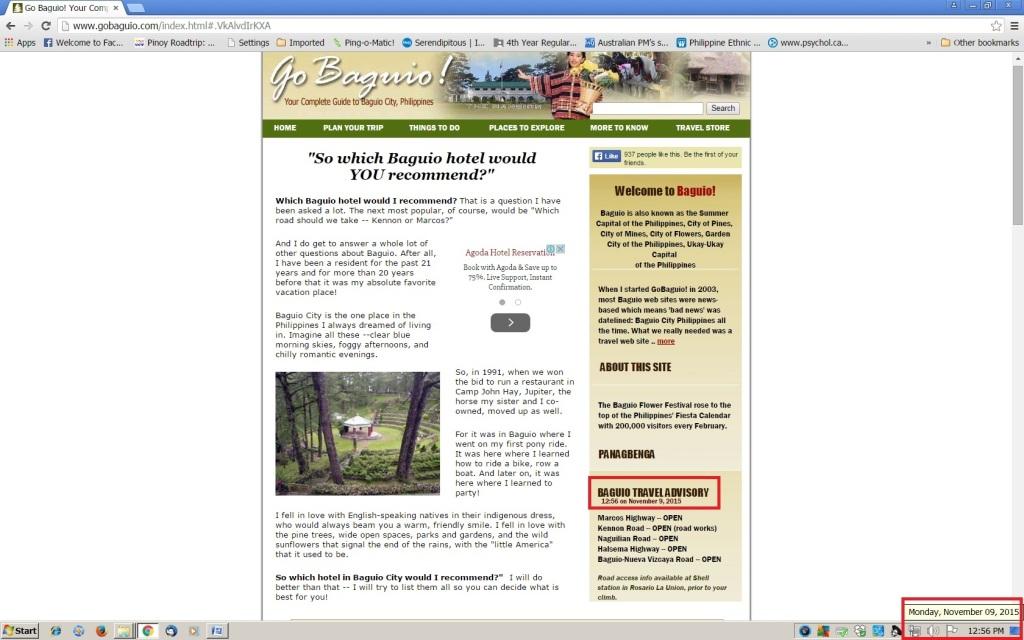This image is a horizontal screenshot of a web page with a predominantly white background. Central to the page is an advertisement for the website "Go Baguio." The webpage features a light blue heading bar with an open tab labeled "Go Baguio." The address bar displays the URL: www.gobaguio.com. Below the address bar, there is a section populated with several icons and bookmarks.

A light gray navigation bar can be seen at the bottom of the screen, containing pinned start programs on the lower right corner. Highlighted in a red box on this navigation bar, it states the date and time: Monday, November 9, 2015, at 12:56 p.m.

The website prominently displays the title "Go Baguio, your complete guide to Baguio City, Philippines." At the top of the page, there is a banner featuring an inset photograph of a woman with a drum, adding a cultural touch. Beneath this banner is a search bar for navigating the site.

Below the search bar, an olive green strip with drop-down menus is visible, containing categories labeled Home, Plan Your Trip, Things to Do, Places to Explore, More to Know, and Travel Store.

The main title of the webpage reads "So Which Baguio Hotel Would You Recommend?" indicating the presence of an article written to offer hotel recommendations. Toward the bottom left-hand side of the article, there is a small inset photograph depicting a forest setting with a dwelling in the center of a circular field.

On the right-hand side of the screen, there is a vertical yellowish-brown scroll-down menu, which provides additional information. Within this section, at the lower right-hand portion, "Baguio Travel Advisory" is highlighted in a red border, matching the red border around the date and time in the lower right-hand corner.